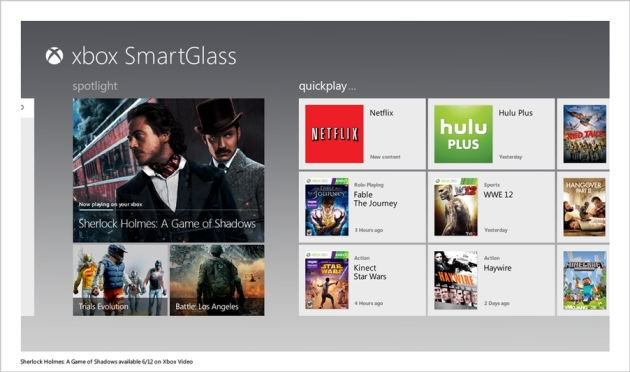In this image, we see an interface of the Xbox SmartGlass application. At the top left, "Xbox SmartGlass" is prominently displayed in white text. The screen is divided into different sections and categories. 

On the left side, the category labeled "Spotlight" features a large thumbnail of the Sherlock Holmes movie "A Game of Shadows." The thumbnail showcases a man in a black suit with longer black hair, standing next to another man in a gray suit, brown hat, and a mustache, against the backdrop of what appears to be a train.

Below the "Spotlight" section, the titles "Trials Evolution" and "Battle Los Angeles" are displayed.

On the right side of the screen, under the title "Quick Play," we see six neatly arranged categories displayed in white squares, separated by two vertical and two horizontal gray lines. From top to bottom, the first column includes:
- Netflix
- Fable: The Journey
- Kinect Star Wars

In the same manner, the second column includes:
- Hulu Plus
- WWE '12
- Haywire

To the right of this, there are three movie covers partially visible, but the titles are out of the frame.

The background of the image is a gradient gray, starting much lighter at the bottom and blending into a standard gray hue towards the top.